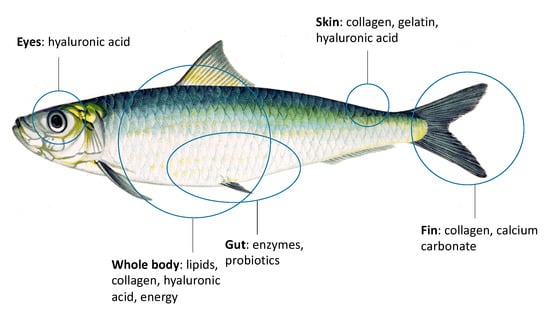The image showcases a hand-drawn fish at the center of a white background, intricately detailed with various annotations. The fish features a striking bluish-green gradient of scales along its back, which transitions to greener hues as it approaches the white belly. Surrounding the fish are a series of circles that direct attention to specific areas, each connected to labeled sections with in-depth information. For instance, a blue circle around the fish's eye leads upward to a label reading "eyes, hyaluronic acid." The scales, particularly around the eye, exhibit a silver sheen with some greenish hues.

The fish's scales are annotated with "skin, collagen, gelatin, and hyaluronic acid," while the midsection is labeled "whole body, lipids, collagen, hyaluronic acid, and energy." The lower fin is indicated with a circle containing the label "guts, enzymes, and probiotics," and another fin includes "collagen, calcium carbonate." The detailed artwork not only highlights the fish’s physical features but also emphasizes various beneficial compounds like collagen, hyaluronic acid, enzymes, and probiotics, designed in a visually informative manner. The overall coloration of the fish includes notable silver around the eye and some yellow tints in certain body parts, adding to its vibrant appearance.